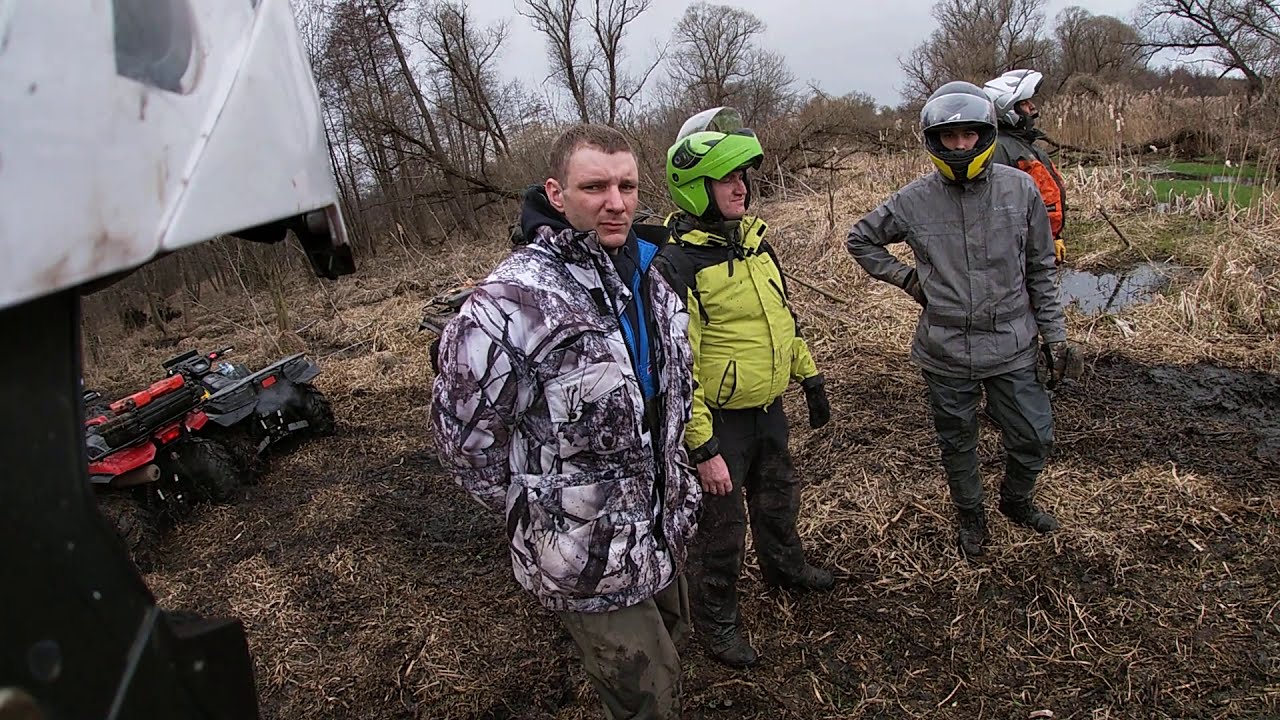The image depicts an outdoor scene featuring five men standing in a barren field beneath a gray, overcast sky. The focal point is a man in a camouflage jacket with a blue shirt underneath, green or khaki slacks, and short brown hair. He has his hands behind him and is positioned centrally. Flanking him is a person in a yellow and black long-sleeve jacket, wearing black pants, black shoes, and a green helmet with the visor up, who has one glove on. Facing the camera is a skinny individual in a dark gray, long-sleeve jacket, gray pants, and dark shoes, accessorized with gloves and a helmet—yellow at the bottom and gray at the top. Further in the background, a person in an orange and black coat with a white helmet looks off into the distance. The field they stand in appears covered with dead leaves or pine straw, with large trees with bare branches framing the image. In the left upper corner, a building or trailer and some ATVs are visible. The overall setting underscores a dormant, wintry landscape.